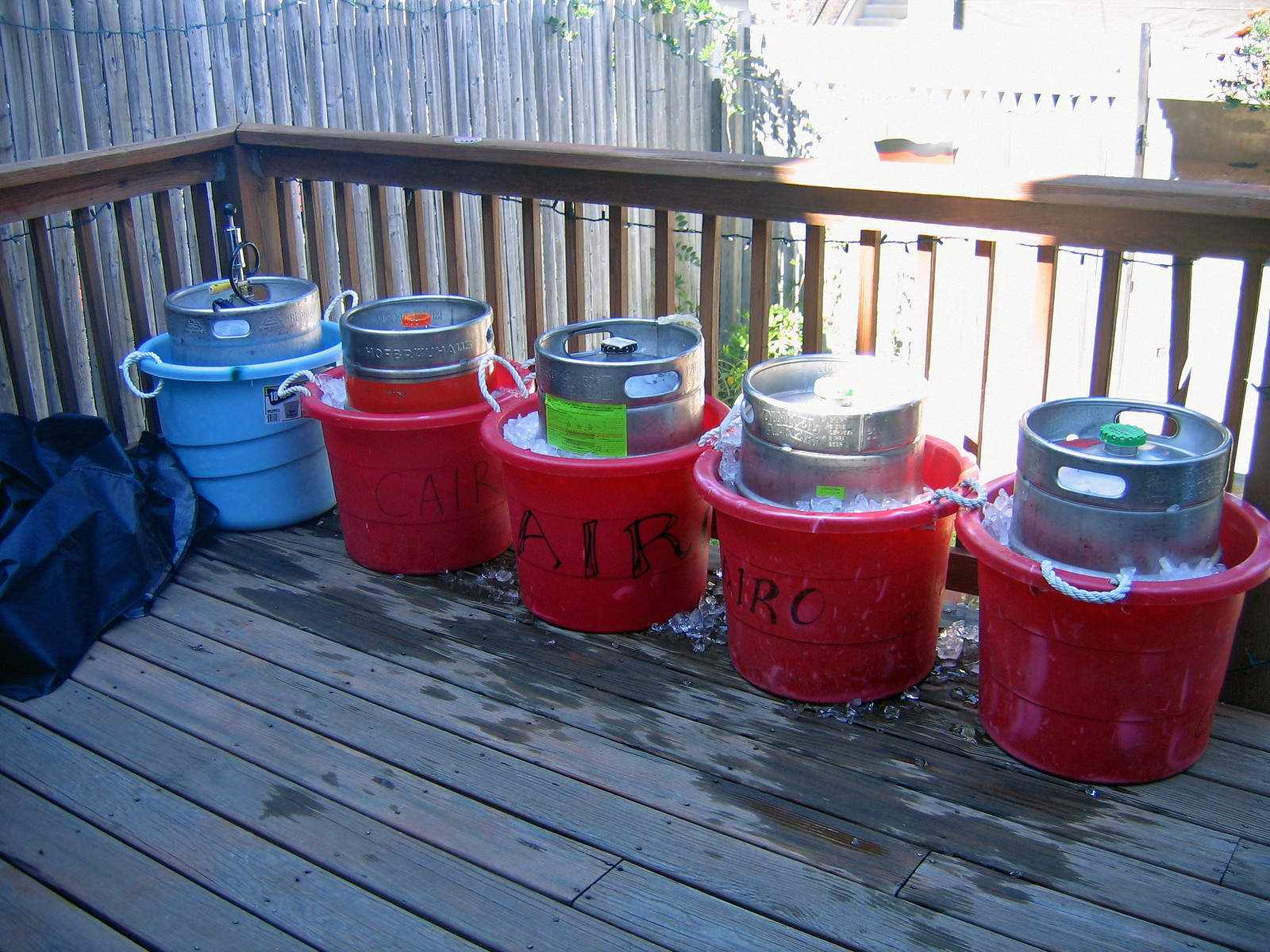The photograph captures a sunlit wooden deck in someone's backyard, bordered by a tall wooden fence. The deck boards, medium-toned and facing roughly 10 o’clock, form the base for a row of five plastic tubs each holding a beer keg. Located near the fence, these tubs are filled with ice, except the one on the far left, which is blue and appears untapped. The other four tubs are red, most displaying the word “Cairo” in black marker. The image is bright, with sunlight making parts of the scene, especially the top right corner, hard to see. The kegs, large aluminum steel canisters standing up to 3 feet tall, weigh around 50 pounds when full.